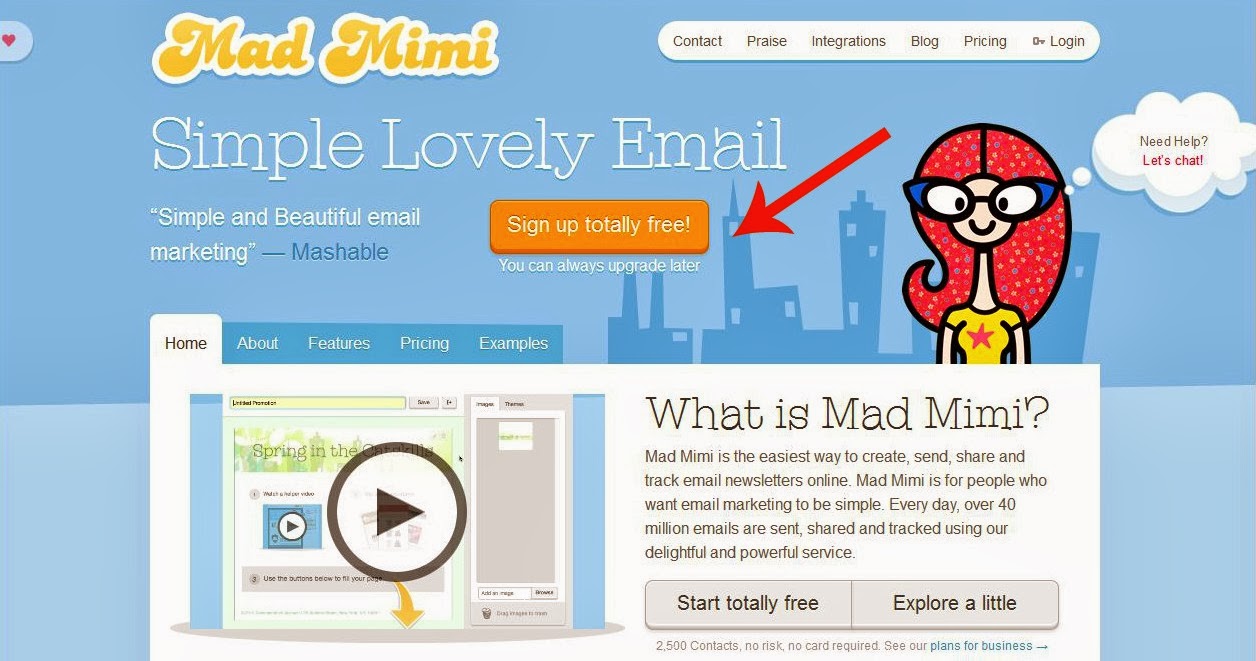The image features a gradient background, transitioning from a darker blue at the top to a light blue at the bottom. On the center right, a skyline of buildings is illustrated in a dark blue hue. Occupying the upper left corner, the text "Mad Mimi" stands prominently in yellow with a white outline. Adjacent to this text, a series of tabs titled "Contact," "Praise," "Integration," "Blog," "Press," and "Login" are displayed against a white background with black lettering.

Below the “Mad Mimi” header, white text reads, "Simple lovely email. Simple and beautiful email marketing. Mashable." An orange button to the right bears the inscription, "Sign up. Socially free." Positioned beneath this section, smaller text reassures, "You can always upgrade later."

In the bottom left corner, there are tabs for navigation: "Home," "About," "Features," "Pricing," and "Example." The "Home" tab is highlighted in white, while the others remain blue. Behind this navigation bar, a video is playing, featuring a play button.

Adjacent to this video, a text block in the middle of the image explains, "What is Mad Mimi? Mad Mimi is the easiest way to create, send, share, and track email newsletters online. Mad Mimi is for people who want email marketing to be simple. Every day over 40 million emails are sent, shared, and tracked using a delightful and powerful service." Below this explanatory text are two grey buttons labeled "Start socially free" and "Explore a little." At the very bottom, it states, "2500 contacts, no risk, no card required, see our plans for business."

Finally, an illustrated character with red hair, donning a yellow t-shirt featuring a red star, is situated toward the bottom. A speech or dot bubble next to the character reads, "Need help? Let's chat."